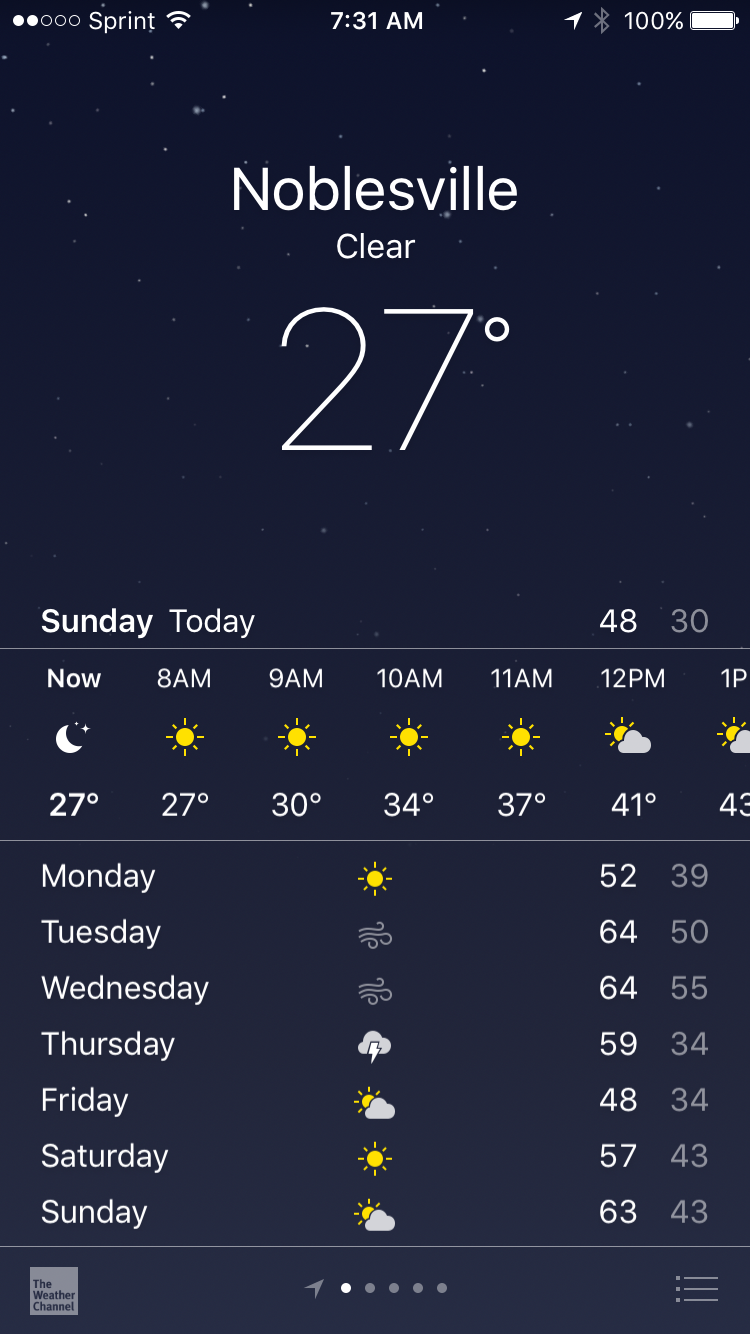A detailed image description of someone's smartphone screen displaying a weather application. The entire background is black, with five small dots at the very top; two of these dots are white while the remaining three are black. The upper left corner of the screen displays the word "Sprint" next to a connectivity icon. Centered at the top, it reads "7:31 AM," accompanied by various icons and a battery indicator showing 100% charge.

In the upper middle section, the screen indicates the location as "Noblesville," with the current weather condition described as "clear" beneath it. In large font, the temperature is prominently displayed as "27 degrees." Below this, the app presents an hourly weather forecast. Further down, a weekly weather report is provided, with days of the week listed—Monday through Sunday—showing the high and low temperatures for each day, as well as weather icons depicting the expected conditions.

At the very bottom left-hand corner, there's a gray box containing an icon and black text that reads "The Weather Channel." Near the bottom of the screen, a set of navigation dots indicates that the display is on the first screen.